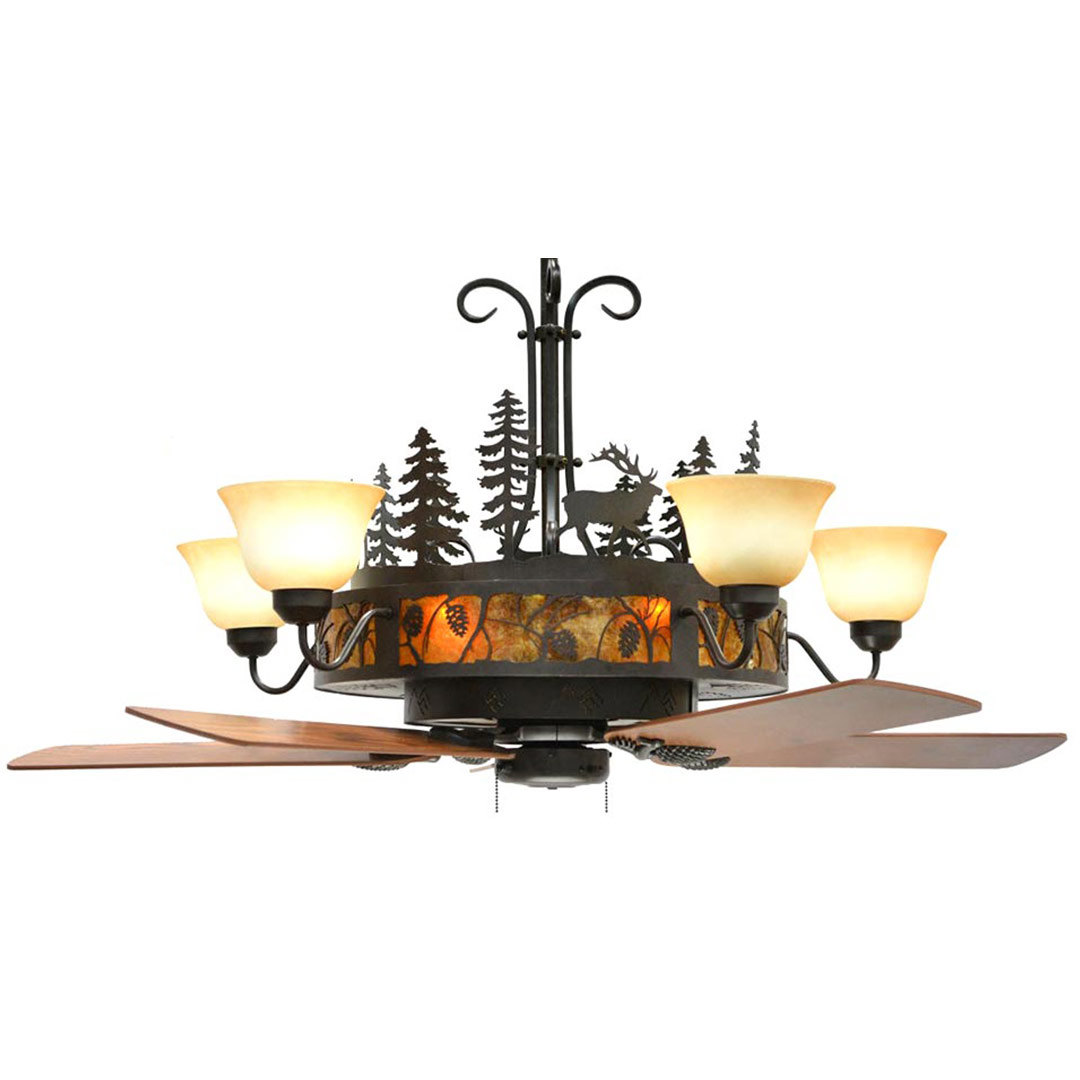The image captures a full-color photograph of an ornate indoor ceiling lamp and fan, illuminated by artificial light. The background is a stark white, likely from a computer screen. The main focus is the detailed ceiling fixture which combines a chandelier and fan, designed with a captivating mix of browns, oranges, and whites.

The fan has four wooden paddles and is equipped with black pull cords hanging from a black motor at the bottom. Above the fan, the light fixture features intricate designs, including metallic pine trees and several moose or reindeer motifs. The base of the chandelier is adorned with black and orange stained glass, forming a visually striking pattern of tree branches and leaves. 

Four upward-pointing lights with white or yellowish shades, reminiscent of tulip flowers, encircle the chandelier. These shades are supported by black fittings that integrate seamlessly into the chandelier's elaborate structure. The handle, or stem, leading up to the ceiling is black and offers a touch of elegance with ornamental curls on either side, completing the exquisite and festive appearance of this unique ceiling fan and lamp combo.